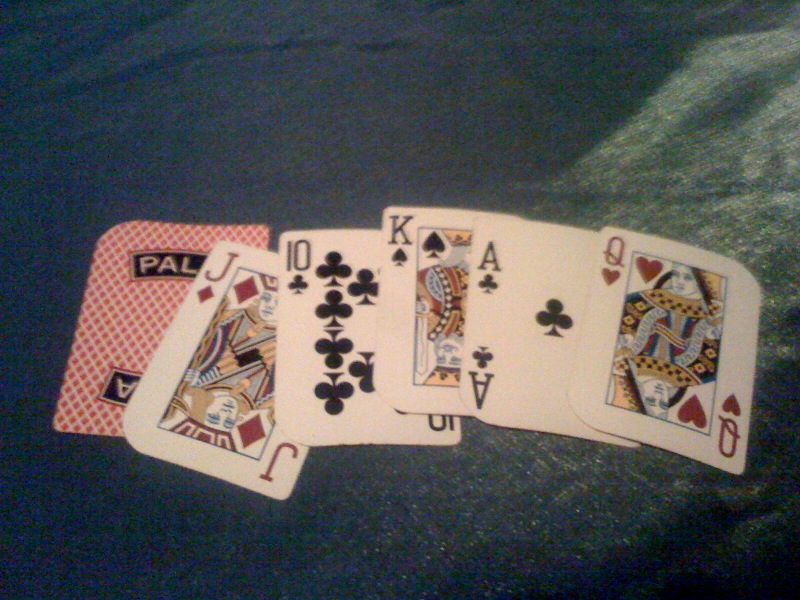An array of playing cards is meticulously arranged in the photograph. The selection includes a Joker card, the Ten of Clubs, the King of Spades, the Ace of Clubs, and the Queen of Hearts. The cards are displayed in a balanced and visually appealing manner, showcasing the distinct designs and suits. The Joker card stands out with its vibrant and intricate artwork, while the other cards present a contrast with their traditional playing card aesthetics. The combination of different suits and values offers a captivating glimpse into the world of card games and the rich history of these timeless objects.